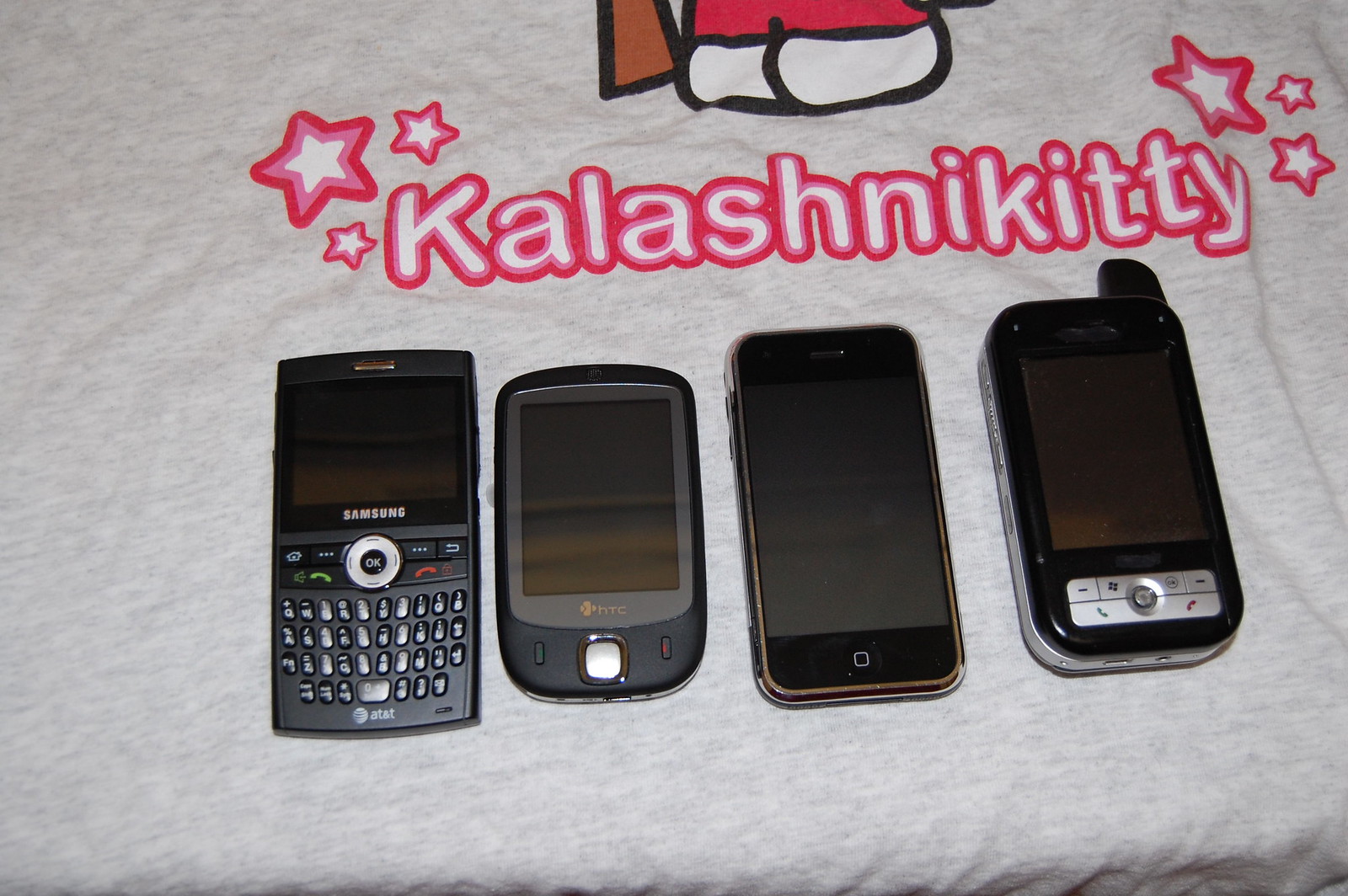The photograph features four older cell phones displayed on a large, slightly wrinkled gray t-shirt. Above the phones, the shirt prominently displays the text "Kalashini Kitty" in white lettering with pink trim, surrounded by three stylized stars in white with multiple pink outlines varying from light to hot pink. The design also includes a partial cartoon image depicting white feet, a brown object, and pink accents, which are all outlined in black. The four phones, from left to right, include: an old Samsung model with a physical keyboard on the front and an AT&T logo at the bottom, an HTC smartphone with a small touchscreen and physical green and red buttons for picking up and hanging up calls, an early model iPhone, and a less identifiable smartphone with physical buttons, possibly a slider type, featuring traditional green and red call buttons. The phones are mostly black with some silver elements.